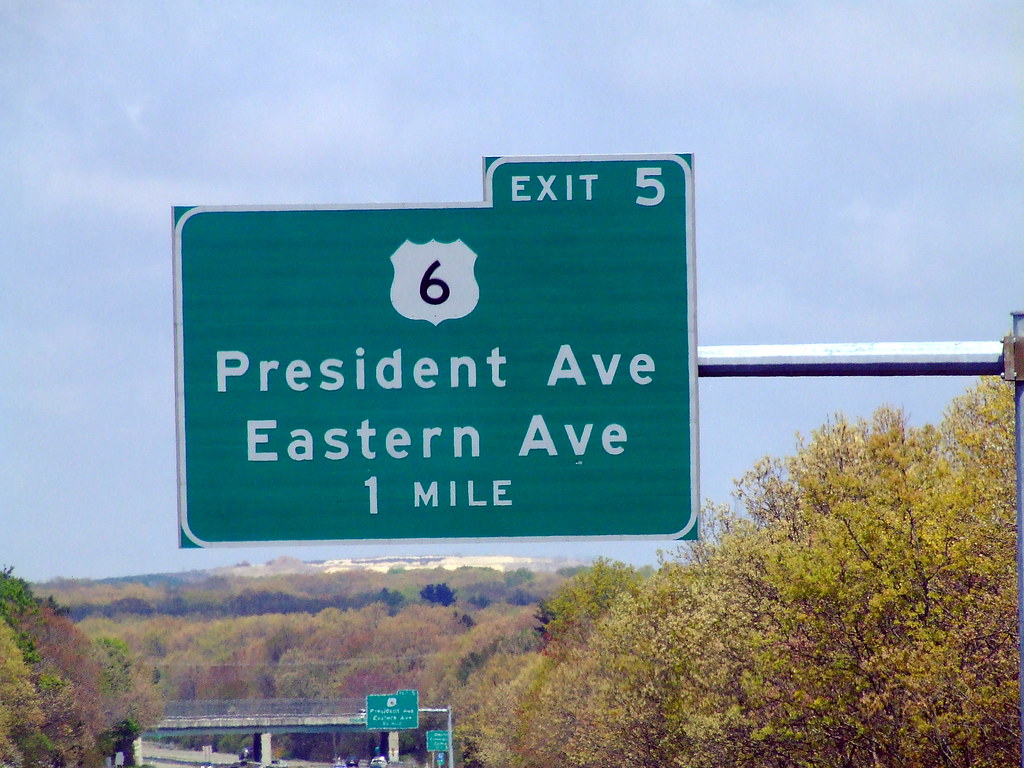The image vividly captures a freeway exit dominated by a large, green rectangular highway sign with a white border. Positioned prominently at the top right, the sign indicates "Exit 5" and features a white shield symbol emblazoned with the number 6. Below, white text provides directional information, stating "President Avenue, Eastern Avenue, 1 mile." The sign looms over the freeway, with another green freeway sign visible in the background indicating the next exit is half a mile away. Below the signage, the freeway stretches into the distance with minimal visibility of the road itself, revealing just the tops of a couple of vehicles. Lush trees frame both sides of the freeway, their foliage displaying a palette of green, yellow, and red hues, suggesting the onset of autumn. The scene is bathed in bright sunlight with a clear, light blue sky punctuated by sparse, wispy white clouds. In the far distance, some white buildings can faintly be seen, adding a hint of human infrastructure amidst the natural landscape.